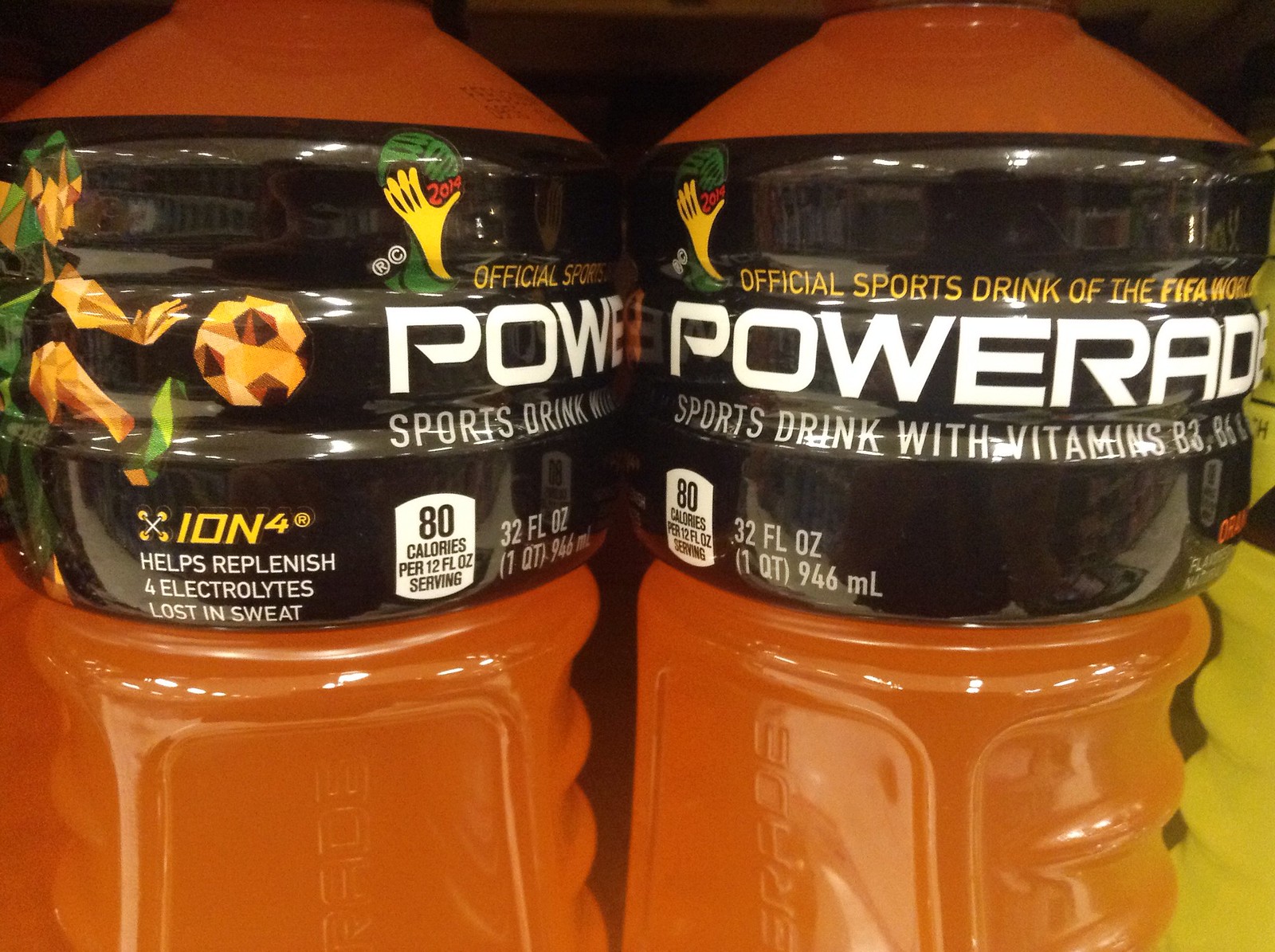The image showcases an up-close view of two clear plastic bottles of orange Powerade. The vibrant orange liquid fills each bottle, which holds 32 fluid ounces (1 quart or 946 milliliters). The label, occupying the upper third of the bottle, is predominantly black with the brand name "Powerade" prominently displayed in bold white letters. Beneath the brand name, the label provides additional details: "Sports Drink with vitamins B3, B6," although the description of the third vitamin is obscured. The label also notes the caloric content of 80 calories.

Above the brand name, a smaller text reads "Official Sports Drink of the FIFA World," but the subsequent text is not fully legible. On the left side of the label, there is a yellow symbol of a hand holding a green object, accompanied by the year "2014."

The bottle on the left features a more distinct image of a soccer player wearing green shoes, green hair, and a green uniform, engaging with a soccer ball. The player, who appears to be light-skinned and of Asian or Caucasian descent, is depicted with a dynamic pose, emphasizing the athletic theme of the product.